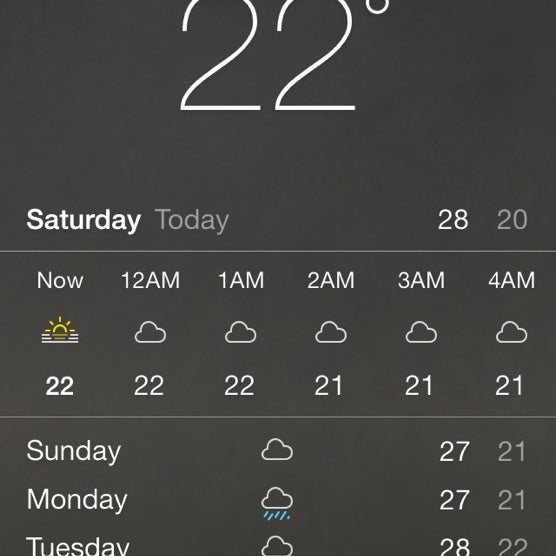A detailed screenshot of a smartphone weather app, likely from an iPhone. The interface primarily uses gray and white text, with some elements in darker gray. At the top edge of the screen, partially obscured, the temperature reads "22°," although the tops of the digits and degree symbol are cut off. Below this, the current day, "Saturday," is displayed prominently, with "today" in gray text beneath it. The screenshot spans several days: Saturday, indicating the 28th, through the next few days.

The weather forecast shows:
- **Saturday:** Partly sunny, currently 22°C. 
- **12:00 AM:** Cloudy at 22°C 
- **1:00 AM:** Cloudy at 22°C 
- **2:00 AM:** Cloudy at 21°C 
- **3:00 AM:** Cloudy at 21°C 
- **4:00 AM:** Cloudy at 21°C 
- **Sunday:** Cloudy, high of 27°C, low of 21°C
- **Monday:** Rainy, high of 27°C, low of 21°C
- **Tuesday:** The forecast is partially cut off, but a cloud icon is visible suggesting cloudy or rainy weather; high of 28°C, low of 22°C.

The uniform design and layout suggest that this is from the default weather app on an iPhone.